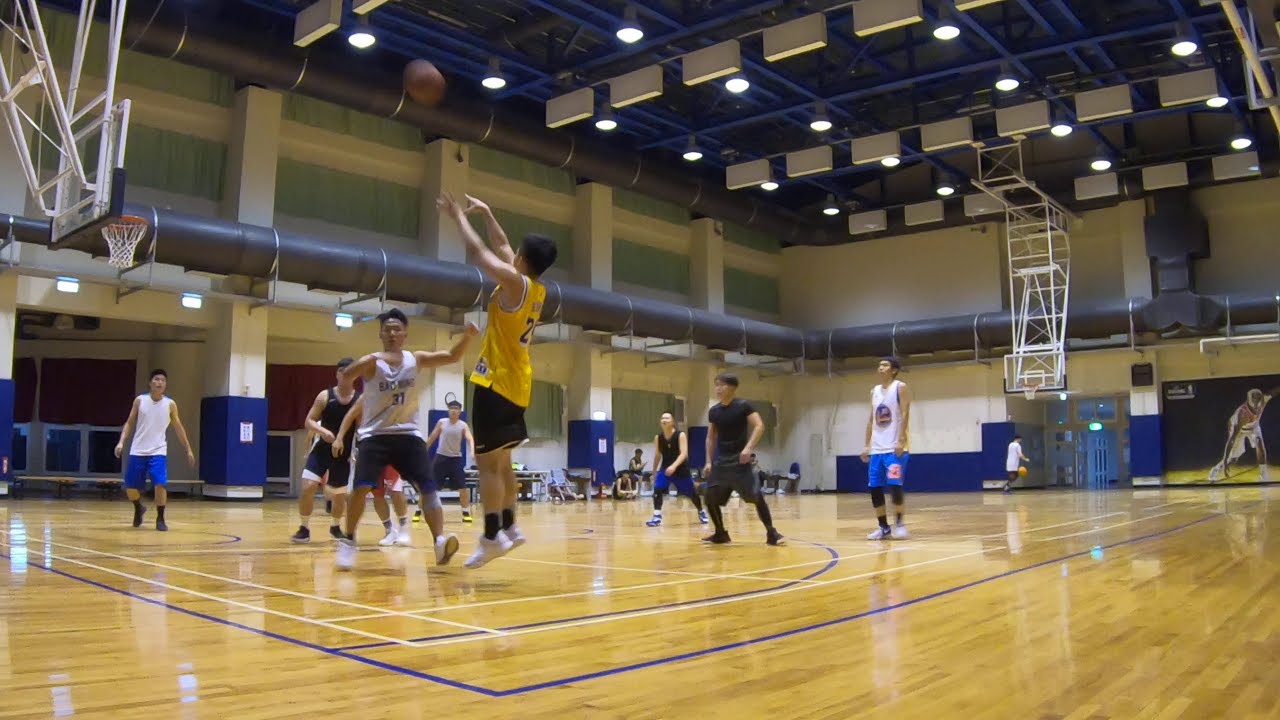In this horizontally aligned indoor scene of a large gymnasium, several players are actively engaged in a casual basketball game. The floor of the gymnasium is a light wood color accentuated with blue and white lines that outline the court. The walls are predominantly white with blue trim at the bottom, housing white columns with blue bases. On each end of the court, there are basketball hoops, and overhead lighting along with exposed pipes gives the setting an industrial look. The players sport various attires, including black shirts, white sleeveless shirts with blue shorts, and a notable player in a yellow jersey and black shorts who is captured mid-air, throwing the ball to another player. In the far background, some spectators are seated on benches and on the floor, engrossed in watching the game. Additionally, a large poster depicting a basketball player is visible on the right-hand side of the gymnasium.